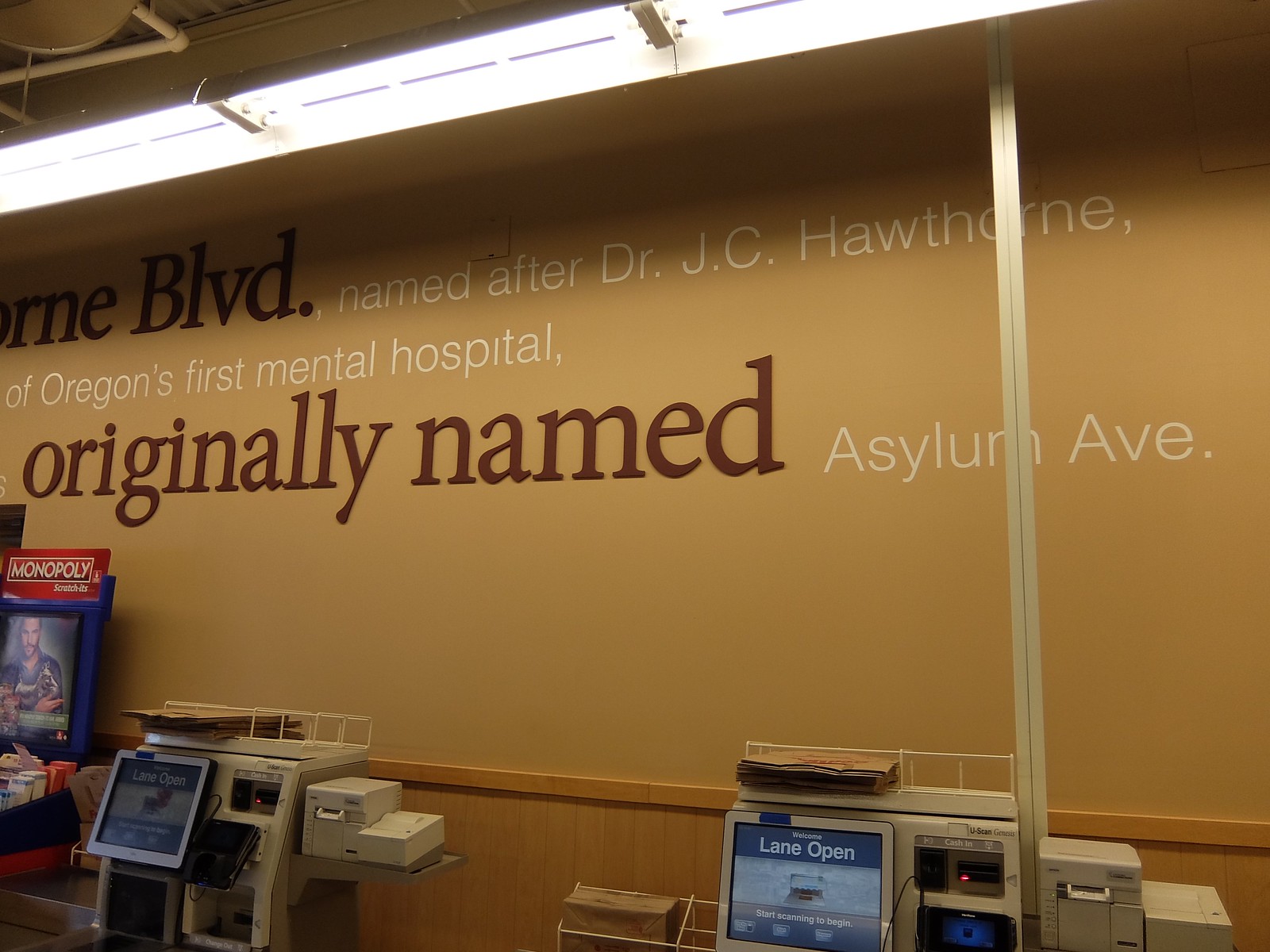The photograph, taken indoors, depicts a checkout area of a store. The upper left section of the image shows an orangey-cream colored ceiling that transitions onto an adjacent wall. Stretching diagonally from the upper right to the upper left are elongated fluorescent light bulbs, casting bright illumination throughout the scene. 

The wall below is pale orange with wooden paneling on the bottom half. Adorning this wall is a series of texts in white and black. Prominently, it reads "named after Dr. J.C. Hawthorne of Oregon's First Mental Hospital" and "originally named Asylum Ave" in large lettering.

In the foreground, there are two self-service checkout machines. Each machine, clothed in a light brown hue, features a screen that displays "Lane Open" on a blue background, and is accessorized with brown paper bags placed both on top and at the sides. Towards the right side of the image, partially visible, is a machine that resembles a lottery or gambling terminal, with a red rectangle displaying "Monopoly" in the distinct font of the board game, accompanied by a screen with an image of a man.

A post descends from the ceiling near the right-hand side of the photo, positioned behind one of the checkout machines, adding to the structured layout of the space.